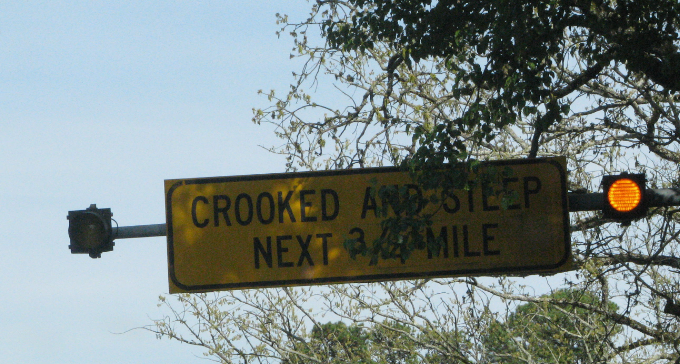The image captures an overhead traffic sign against a backdrop of a very pale blue sky. Surrounding the sign, you can see the tops of large, old trees characteristic of those that grow alongside highways. The sign is mounted on a horizontal pole that spans the road, positioned high above. On the right side of the pole, there's a lit red light, while on the left end, there is another light that presumably turns green. The traffic sign has a white background with a black border and features bold, black capital letters that read: "CROOKED AND STEEP NEXT 3/4 MILE."